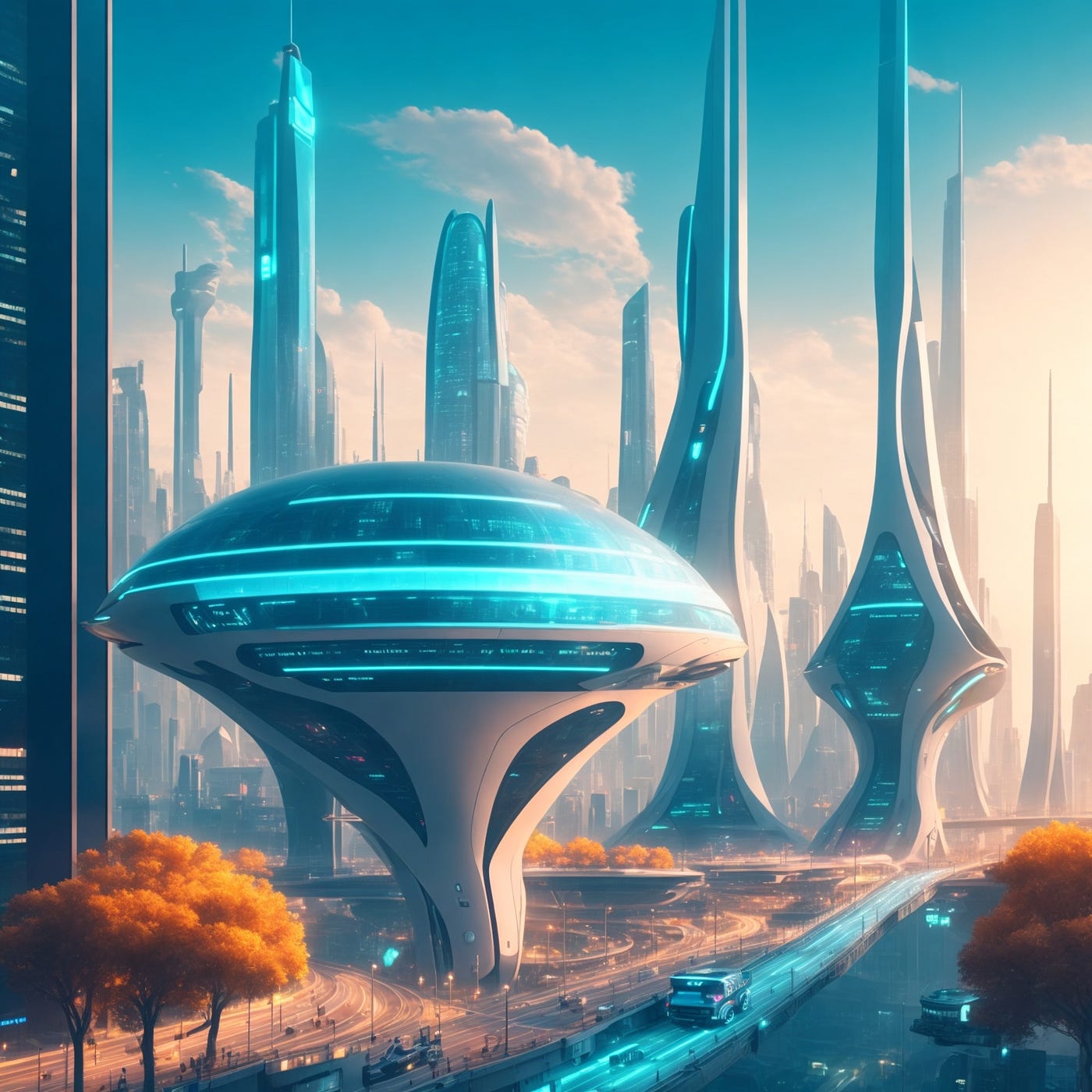The image portrays a highly detailed, computer-generated depiction of a futuristic city under a clear blue sky dotted with white, puffy clouds. Dominating the skyline are sleek, silver skyscrapers with elegant, curved spires that glow with bright blue lights and feature dark blue glass windows. Among these, several buildings, reminiscent of those in Dubai, exhibit twisty and unusually tall, yet animated, structures. Off to the left edge is a particularly tall, rectangular building that stretches out of the frame.

In the foreground, a prominent and distinctive mushroom-shaped building draws attention. This multi-storied structure has a narrow, unstable-looking base that blooms out into a large, clear glass dome adorned with blue lights and intricate line patterns.

On the ground level, there is a narrow highway running through the scene, surrounded by streetlights, and both blue and orange trees, some with yellow leaves, adding vibrant colors to the setting. A large vehicle, serving possibly as a bus or armored transport, moves along the thoroughfare illuminated by the city’s characteristic blue lights.

Overall, this digital artwork captures a sophisticated, sci-fi vision of a future Earth, emphasizing advanced architecture and a harmonious blend of nature and urban elements.